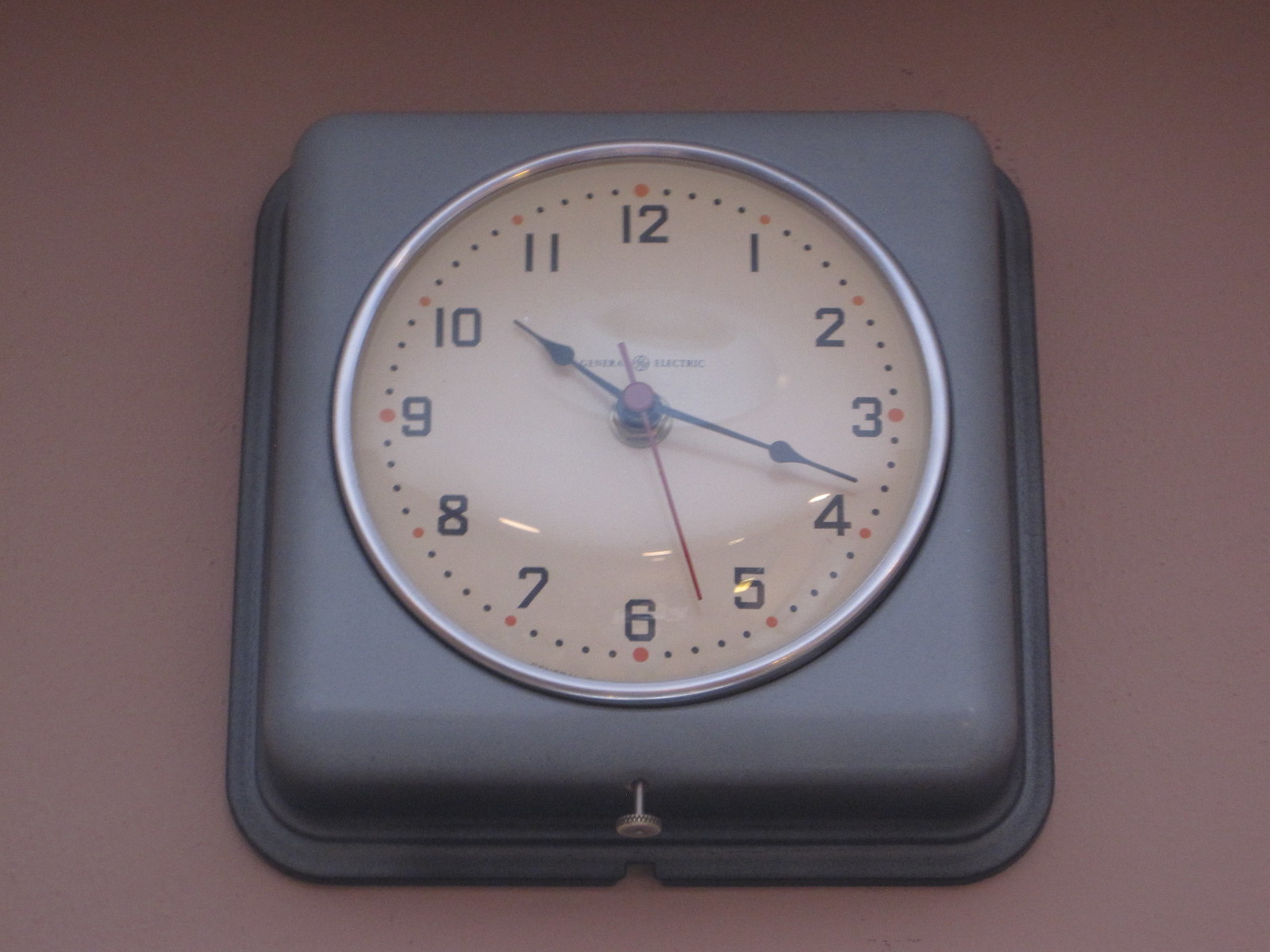In the image, a wall clock is mounted on a pink, slightly faded wall. The clock is encased in a cool gray, metallic square housing that resembles an upside-down plastic tub or baking dish. The clock face is off-white, possibly discolored with age, and is framed by a bright silver rim. The clock features black Arabic numerals from 1 to 12, with orange dots marking each hour and additional black dots around the clock. The General Electric name is faintly written in the middle of the clock face. The time displayed is 10:18, with black hour and minute hands, and a red second hand. A small silver adjustable dial for changing the time is located underneath the frame.